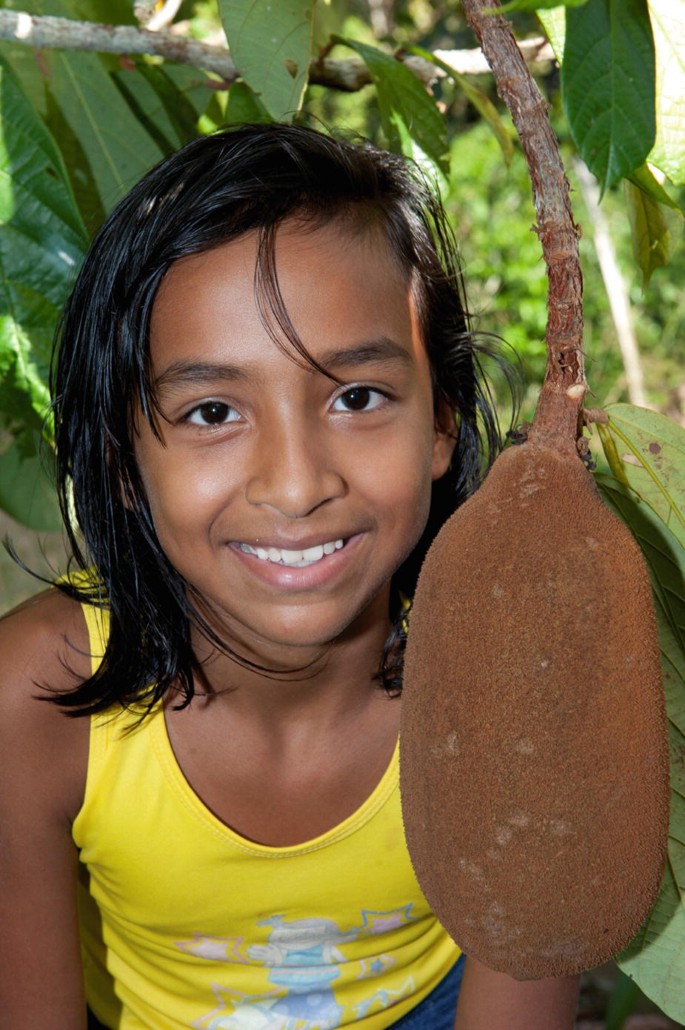In this vibrant portrait, a young girl with tanned skin and long, dark, straight hair stands out against a sunny, lush island backdrop. She wears a bright yellow tank top adorned with a white and blue cartoon design, paired with blue shorts. The girl smiles warmly at the camera, her dark eyes shining with joy. To the right, a tree branch prominently features a large, brown, fuzzy fruit that resembles a coconut, hanging directly in front of her. The background is filled with abundant green leaves and foliage, denoting a tropical or beach environment bathed in bright daylight.